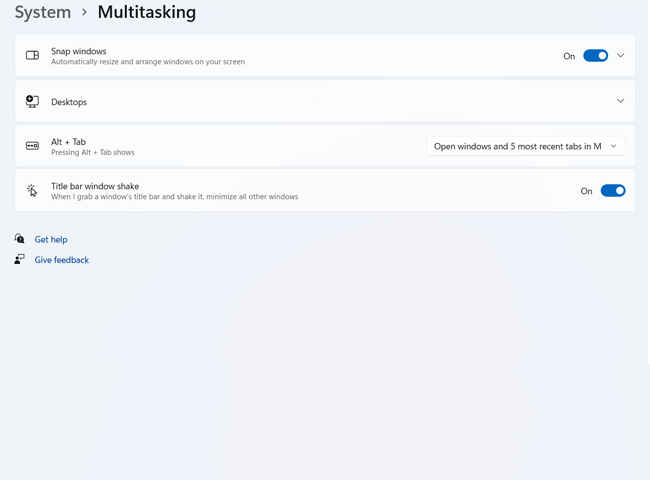This image is a detailed screenshot of a computer settings menu, specifically in the "System" category, showing the "Multitasking" submenu. The main menu item "System" is highlighted in grey and features a grey arrow pointing to "Multitasking," which is listed in black, indicating the current subcategory being viewed.

The primary section is visually framed by a blue border, and the subsequent submenu items are displayed within a white background. To the left, there is an icon of a window next to the label "Snap windows," with a description: "Automatically resize and arrange windows on your screen." To the right of this label, a toggle indicates that the feature is enabled, showing "On" in blue, accompanied by a drop-down menu.

Further down, the menu lists "Desktops," next to a drop-down menu that presently has no selection shown. Below this, a section for "Alt + Tab" is visible, explaining its function: "Pressing Alt + Tab shows," followed by the options "Open windows and five most recent tabs in M," though the full text is truncated. This feature too has a drop-down menu likely containing additional options.

Next, the "Title bar window shake" feature is described with the text: "When I grab a window title bar and shake it, minimize all other windows," and it is turned on, indicated by the selection being in blue.

At the bottom of the menu, which is shaded blue, there are two additional options. The first option, "Get help," is signaled by a chat icon on the left and is highlighted in dark blue. The second option features an icon of a person with a text bubble above their head and is labeled "Give feedback"; this option is also highlighted in blue, but not currently selected.

Overall, the image meticulously details various multitasking settings, providing both textual explanations and visual indicators for each feature’s current status.